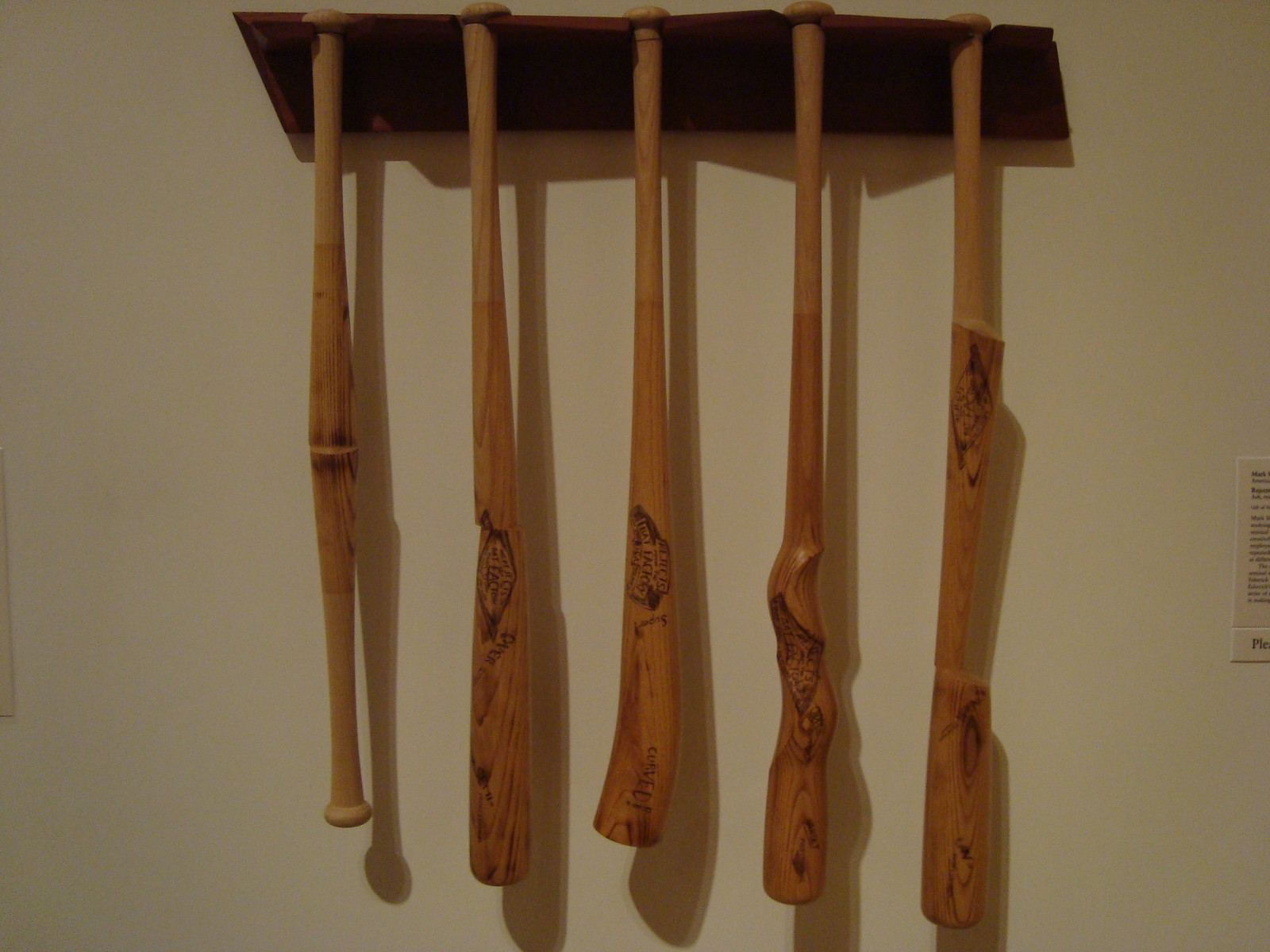This image depicts a collection of five intricately designed wooden bats hanging from a dark brown wooden rack mounted on a wall that appears light beige under the dim lighting. Originating as baseball bats, with one resembling a typical cricket bat, these bats vary dramatically in style. Each bat showcases an unconventional design: one resembles a baseball bat while others are creatively carved into shapes like a machete, a toy rifle, and one with dual handles. The wood grain texture is distinctly visible across all the bats, suggesting artisanal craftsmanship. A portion of a partially visible sign on the right hints that this unique display, likely in an art gallery or museum, is intended to examine the intersections of familiar sporting equipment and imaginative artistry.